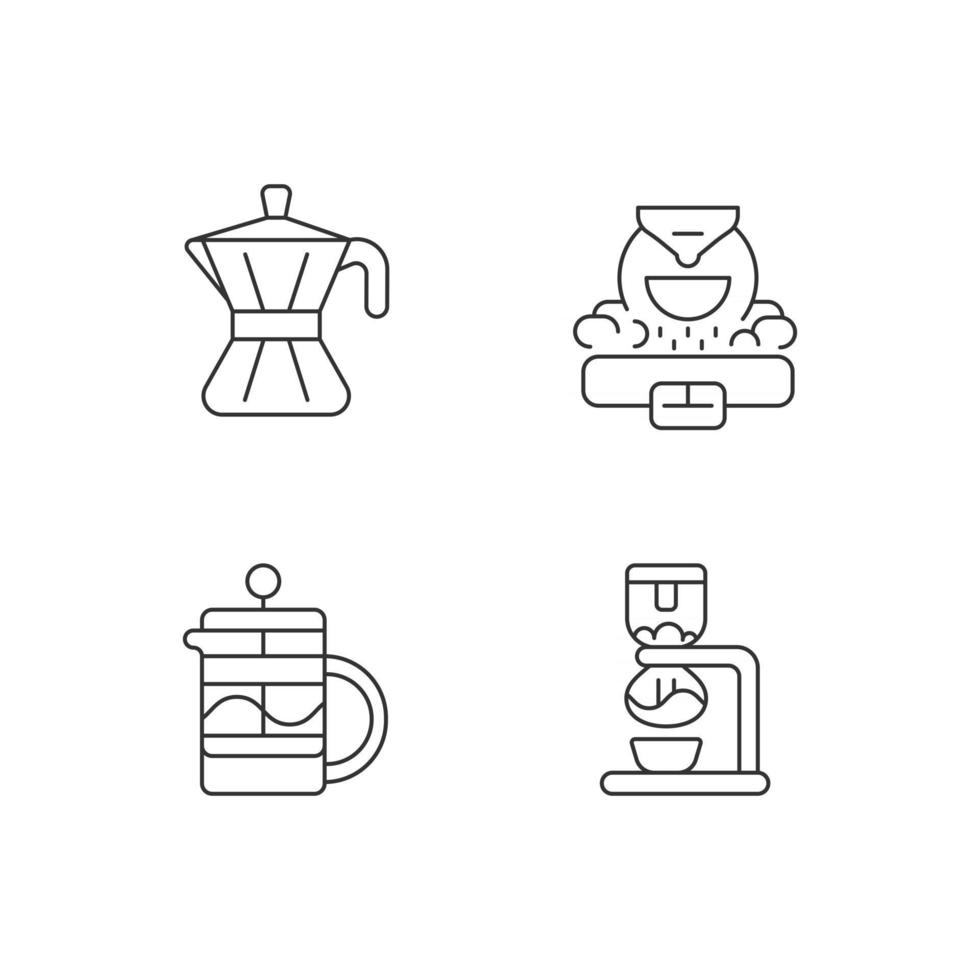This monochromatic artwork comprises four distinct black-and-white illustrations arranged in a square formation. 

- **Upper Left Corner:** A minimalist pitcher is depicted here. It features a handle on the right side and a horizontal line bisecting its body, dividing it into two triangles; the lower triangle is right-side-up, while the top triangle is upside down.
  
- **Lower Left Corner:** This section showcases another pitcher, this time with a more geometric appeal. It has a rectangular body and a circular handle attached to the right side.

- **Lower Right Corner:** Illustrated here is what appears to be a coffee maker. A cup is positioned underneath, suggesting it's ready to brew or dispense coffee.

- **Upper Right Corner:** This section presents a dish, which is visibly surrounded by soap suds, giving the impression of a cleaning scene.

Together, these drawings form a cohesive and detailed representation of common household items, rendered in a simple yet expressive monochrome style.